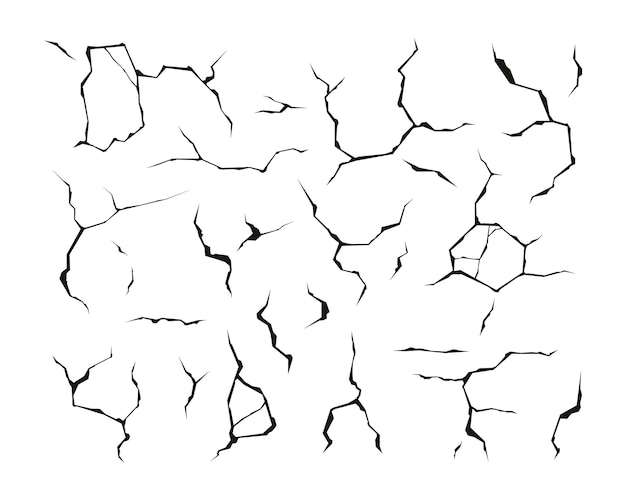The image showcases an intricate network of black cracks sprawling across a plain white background, reminiscent of cracks forming in a pavement after a sharp impact. Starting from the upper left-hand corner, a slightly disconnected crack branches out into a significant rectangular upward crack, which then diverges in various directions. The cracks splinter into an array of unique shapes and patterns, creating a striking visual akin to shattered glass.

Throughout the image, the cracks take on numerous forms—some resemble the letter Y or elongated and reversed letters such as E and M, while others form shapes like hexagons, octagons, and even vague outlines akin to tiny birds. The lower-left crack appears to shape a 'D', while another on the bottom-right takes the form of an 'F'. Despite the diversity in their shapes, the cracks exhibit a certain pattern and organization, contributing to a cohesive, albeit fractured, design.

In total, there are approximately 34 cracks, each diverging in distinct trajectories and sizes. Some cracks are slender and minimalist, while others are robust, appearing as if they spread out from a single point of impact. The intricate interplay of line and form generates a complex, almost chaotic visual texture on an otherwise plain white backdrop.